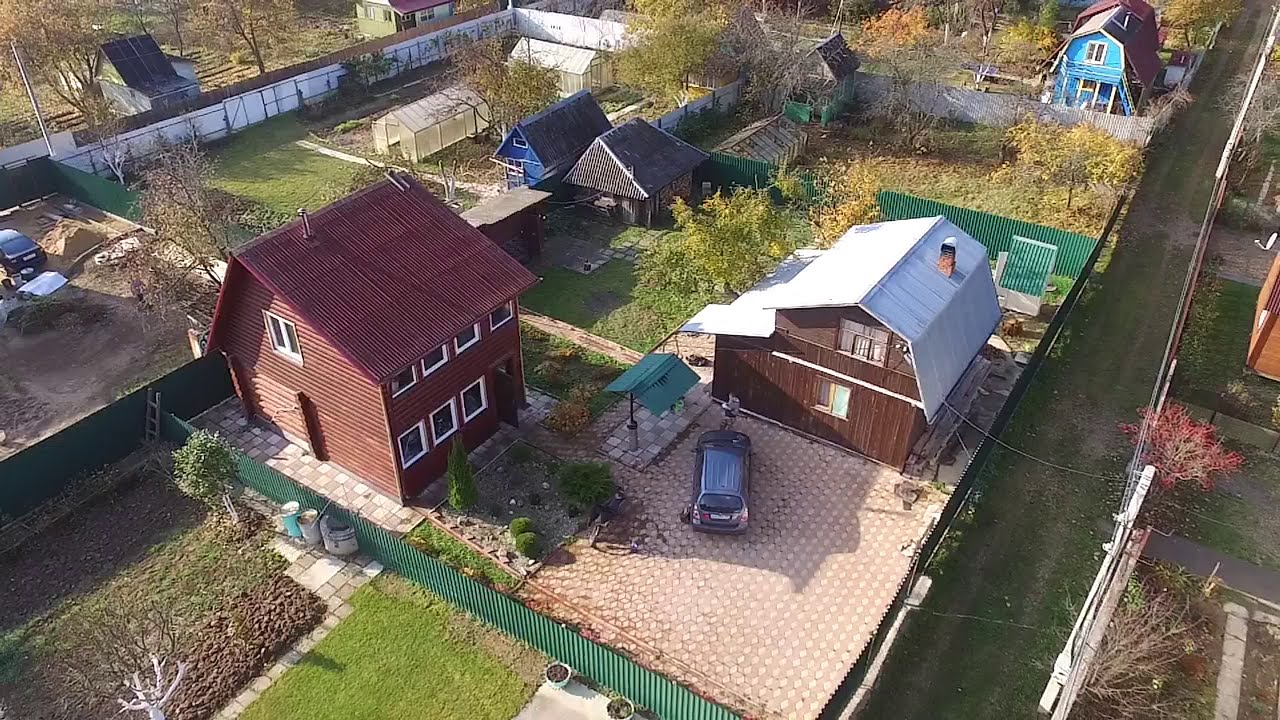This aerial photograph, likely taken from a drone, captures a residential area with various properties and noticeable features. Centrally positioned in the image are two main brown wooden buildings which share a light brown or beige tiled driveway. The building on the left is a two-story structure with a dark maroon, triangular roof and multiple rectangular windows with white frames. Adjacent to this building is a dark SUV parked in the driveway. To the right of the driveway is another wooden building with a silver-colored, metal roof shaped like a barn.

Surrounding these central structures are additional properties and details. Behind and adjacent to these two main buildings is a green yard enclosed by a green fence. Further back, there’s another yard and what appears to be a garden area with patches of dirt and some trees. Towards the top-left, there are two small greenhouses, while to the upper right, a blue house enclosed by a white fence can be seen. The street running parallel to the central structures is paved, and various sections are demarcated by white fences. Overall, the photograph reveals a patchwork of homes, yards, and plots, all arranged within a fenced community, evoking a sense of rural or suburban landscaping, possibly resembling areas found in places like England.